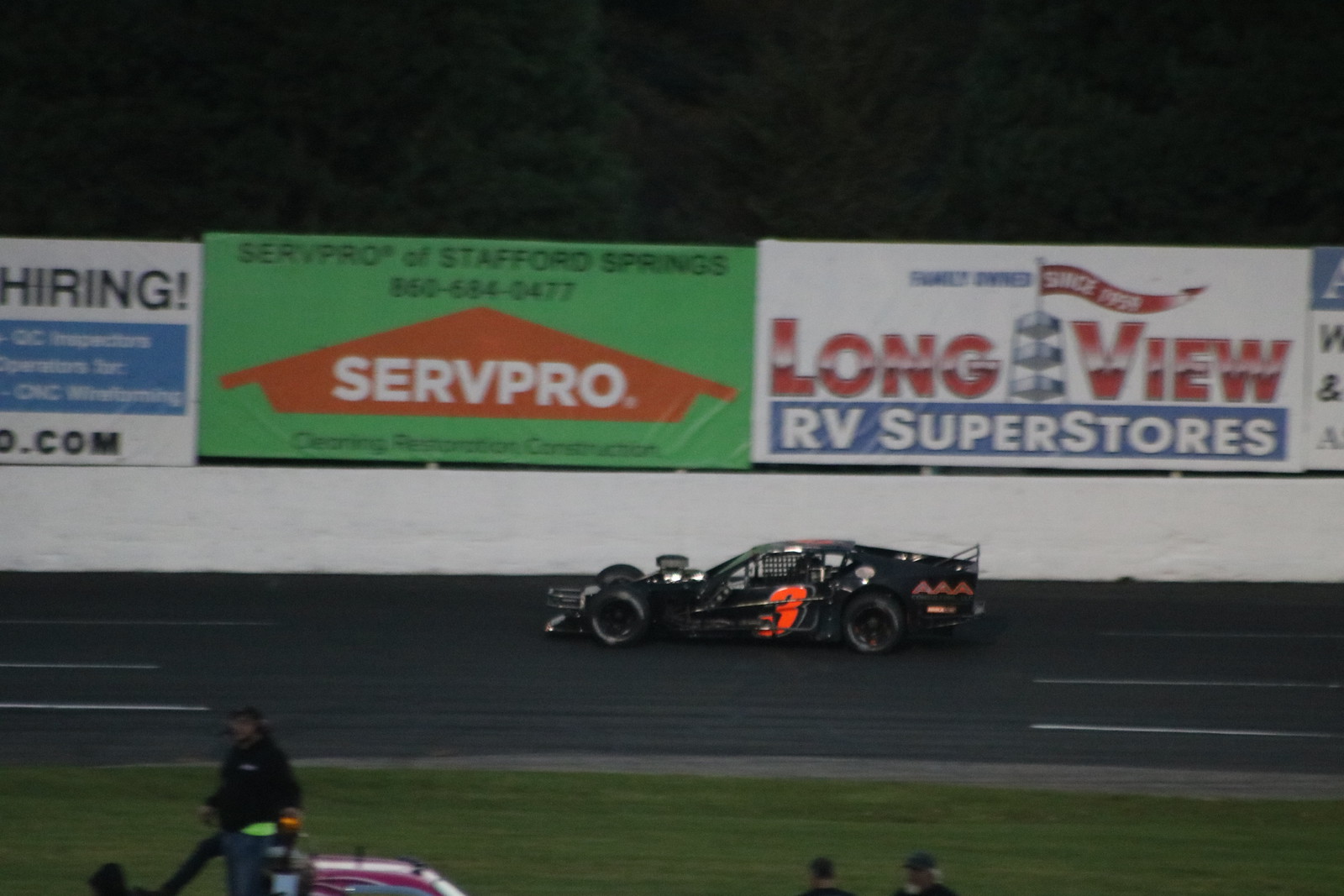The photograph captures a nighttime NASCAR race from a trackside perspective. Dominating the scene is a black race car, identifiable by an orange number three on its side, speeding towards the left. The racetrack, with its three lanes separated by white lines, stretches across the middle of the image. Above the track, a long white crash wall is visible, adorned with several sponsor banners, including notable names like ServPro and Longview RV Superstores. ServPro's banner features a green background with an orange triangle, while Longview's banner includes red lettering. In the foreground, a grassy area stretches horizontally with a pink and white striped truck. Standing in the cab of the truck, a man dressed in a black jacket and jeans appears to be holding a microphone. Nearby, two other individuals, identifiable only by their caps, are also present. The top of the image is bordered by a horizontal black strip, adding to the nighttime ambiance of the scene.